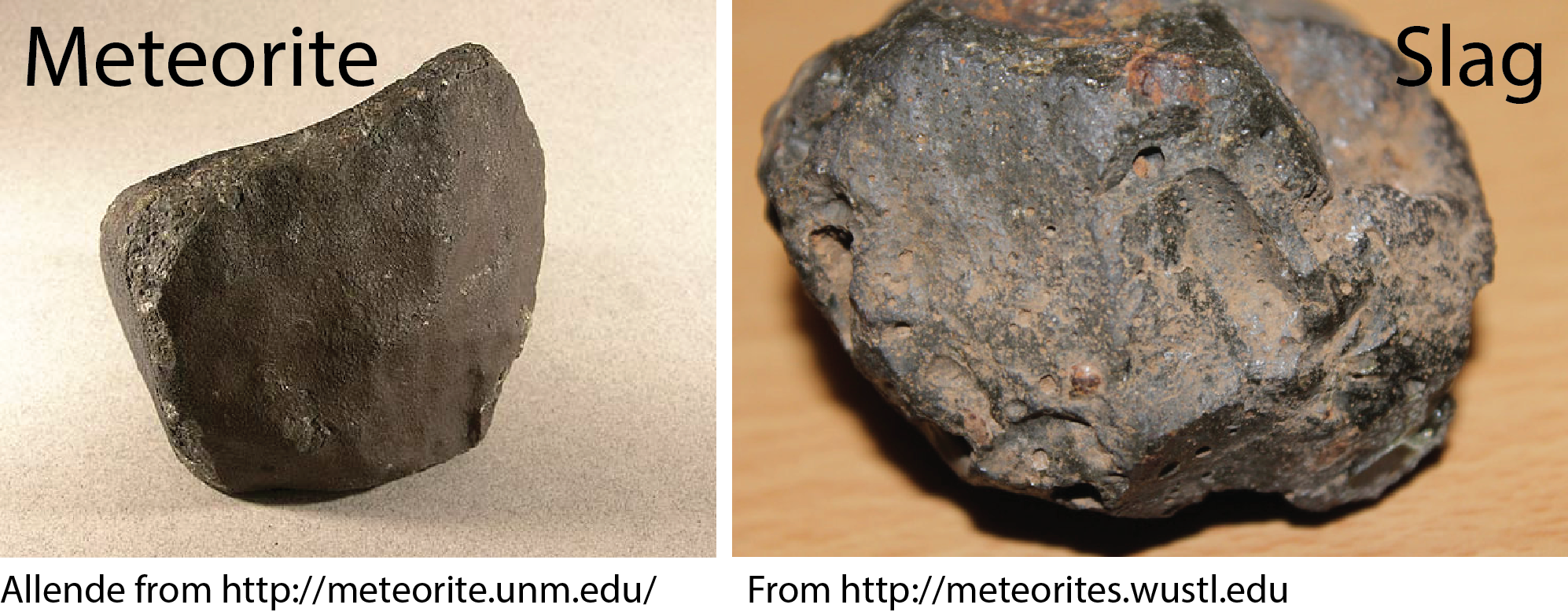The image depicts a comparison between a meteorite and slag, separated into two rectangular sub-images. The left sub-image, set against a light beige background, features a dark gray meteorite standing upright. In the upper left corner, black lettering reads "Meteorite" with a capital M. Below this sub-image, text states "Allende from http://meteorite.unm.edu." The right sub-image showcases a black, round piece of slag lying flat on a light oak surface. The upper right corner of this sub-image contains the word "Slag" in black lettering with a capital S. Below it, a website address reads "from http://meteorite.wustl.edu." The detailed juxtaposition emphasizes educational material, visually comparing the different characteristics and origins of the meteorite and slag.